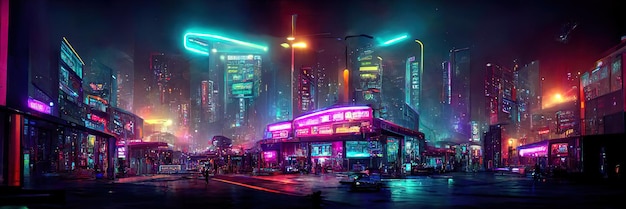The image depicts a detailed, night-time scene of a cyberpunk-styled futuristic city. Dominated by towering skyscrapers in the background, the cityscape is ablaze with an array of vibrant neon lights, primarily in purples, pinks, blues, and some yellows. These lights reflect off the wet streets, adding a shimmering effect that enhances the ambiance. 

In the foreground, there is a small diner adorned with purplish and red neon lights, situated on the corner of a bustling street. The street is lined with various shops, each illuminated by their own colorful neon signs. Orange street lights hang above the different restaurants, adding additional layers of light. 

No people are visible in this particular depiction, though one car and possibly a motorcycle can be seen, contributing to the busy, yet eerily lifeless, urban landscape. The overall dark setting of the city is contrasted by the glow from the neon lights, casting a vibrant, almost dreamlike luminescence across the entire scene. The image encapsulates the essence of a cyberpunk universe, blending elements of modern urban life with a highly futuristic aesthetic.